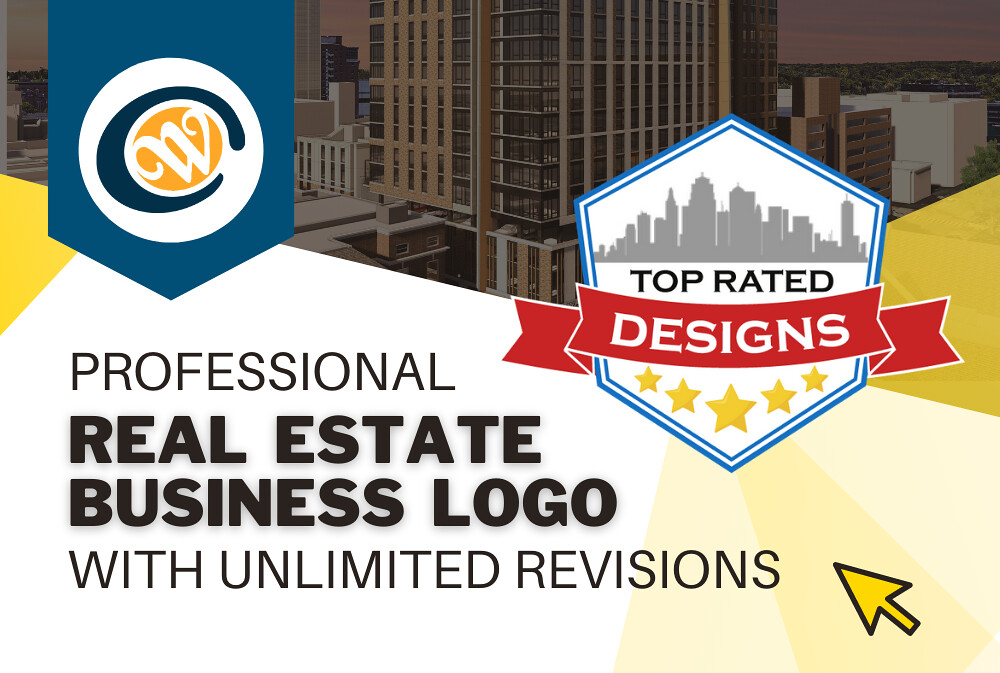This advertisement for a professional real estate business logo service features a visually engaging design dominated by shades of tan, blue, white, red, and yellow. The top section showcases a partial cityscape with tall buildings, including one with prominent brown, light brown, and black beams, hinting at a sunset and greenery in the distance. 

Prominently displayed in the ad are two distinct logos: one is a white circle featuring a stylized W in an egg-shaped golden area with a surrounding blue curve, and the other is a silhouette of distant grey buildings above a banner. The banner, in red with white text, states "Top Rated Designs" flanked by five gold stars, indicating high quality. An eye-catching yellow arrow points up to the left, drawing attention to the text.

In black, the text boldly states "Professional Real Estate Business Logo with Unlimited Revisions," with 'Real Estate Business Logo' in thicker font, emphasizing the service offered. The overall design reflects precision and expertise, aimed at real estate and architectural businesses.